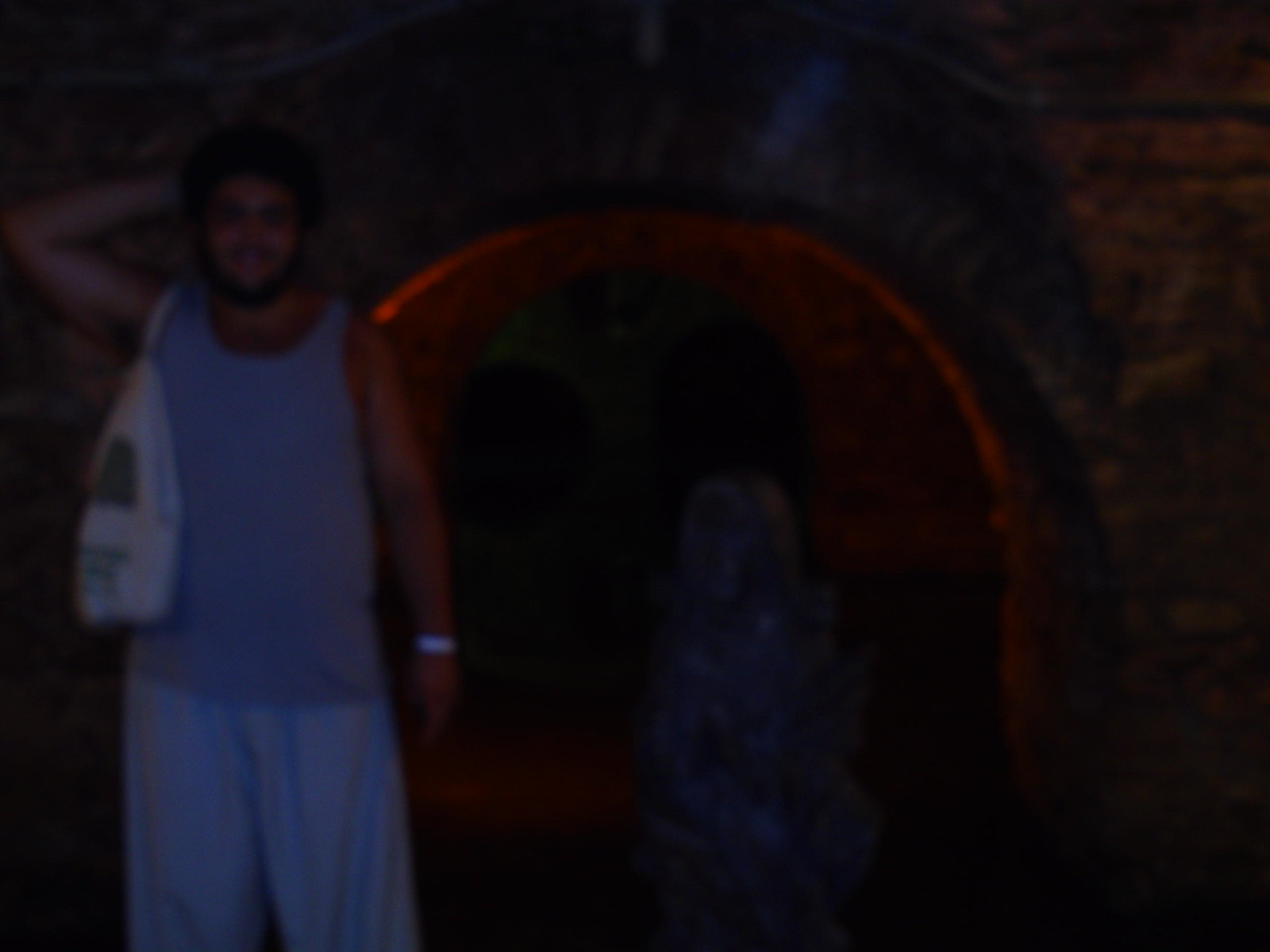The image is a low-quality, blurry, and dark square photograph. Despite the poor resolution, one can discern a person standing on the left side of the frame. The individual has black hair and a beard, and is wearing a grey tank top. A white item adorns his left wrist, and he carries a white bag over his right shoulder. His bottoms are also white. In the background, there is a noticeable red shining light, adding a stark contrast to the otherwise dim image.